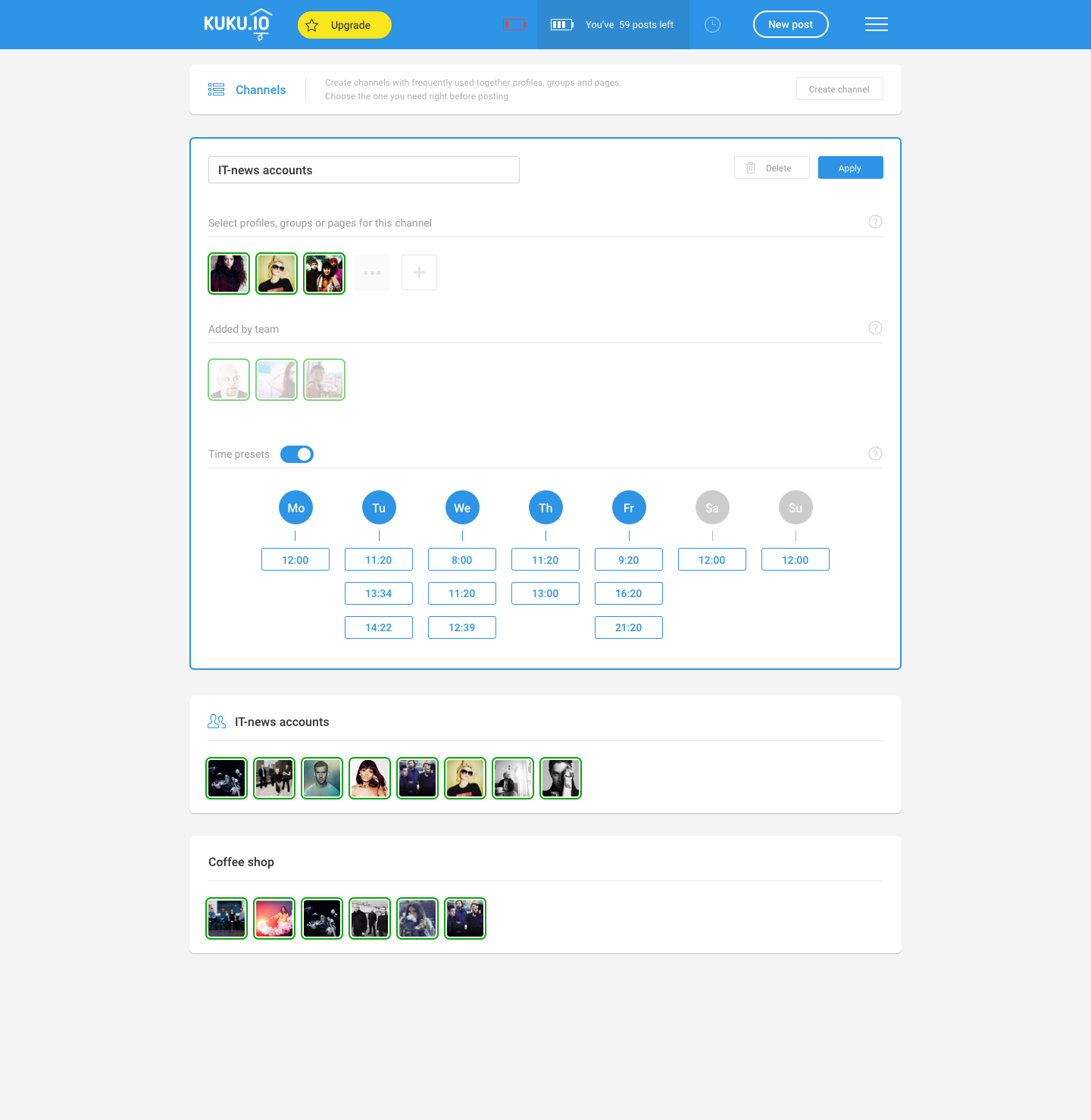Screenshot of a website called Kuku.io, spelled K-U-K-U dot I-O. The top of the screen features a blue bar containing several icons. The first icon is the Kuku.io logo, followed by a yellow button with a star that says "Upgrade" in black text. Next to it is an icon resembling a battery displaying "You've 59 points left." Adjacent to the battery icon is a blue button outlined in white, with white text in the center that reads "New Post." To the right of this button is a hamburger icon consisting of three lines.

Below the blue bar, there is an icon that looks like a list, labeled "Channels." On the right-hand side in grayed text, there is a button labeled "Create Channel." A white-outlined square, which is actually outlined in blue, contains a search bar with the placeholder text "IT-News Accounts." Beneath the search bar, it says you can select profiles, groups, or pages for the channel. 

A series of avatars are displayed for adding profiles. In the upper right-hand corner, there is a blue "Apply" button, with a white "Delete" button situated directly to its left, allowing for the selection and removal of channels or profiles. An option for channels or profiles added by the team is present as well.

Further down, there are columns representing each day of the week, abbreviated from Monday to Sunday, with each column containing various time slots in military time format. For example, Monday has a slot at 12:00, Tuesday includes slots at 11:20, 13:34, and 14:22. Below these time slots, a list of IT-News accounts is displayed.